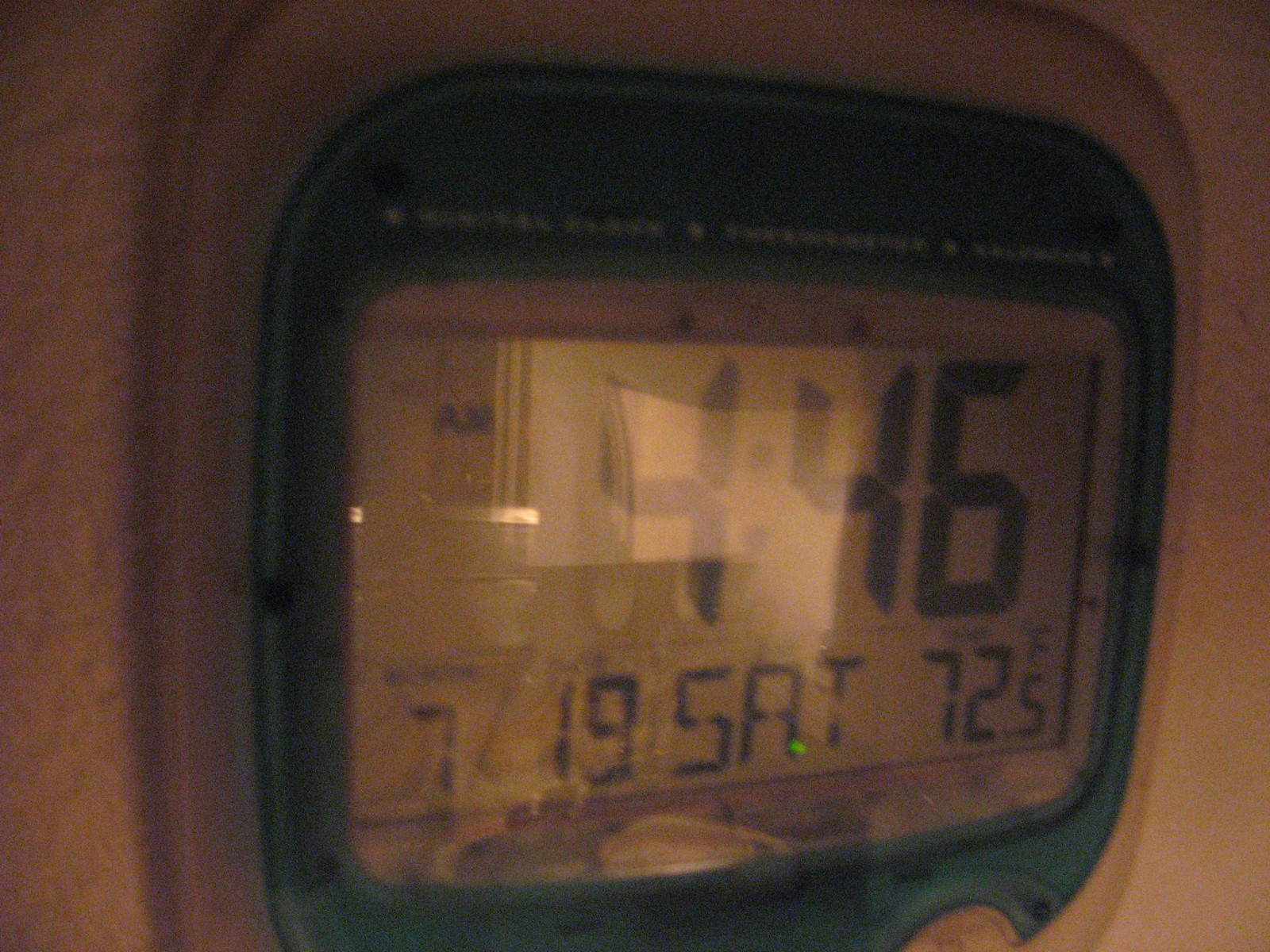This is a close-up photograph of a digital thermostat, housed in a clear cover. The image is dark and somewhat grainy, and there is a notable rectangular white glare at the center of the thermostat's cover. The thermostat's LCD screen displays the time as 4:46 AM and the date as Saturday, the 19th. In the lower-left corner, the thermostat shows the number 7, and in the lower-right corner, it displays the temperature of 72.5 degrees Fahrenheit. The digital screen is surrounded by a dark frame with rounded edges, which is further encased in a lighter-colored frame, also with rounded corners. The thermostat is mounted on a light-colored wall.